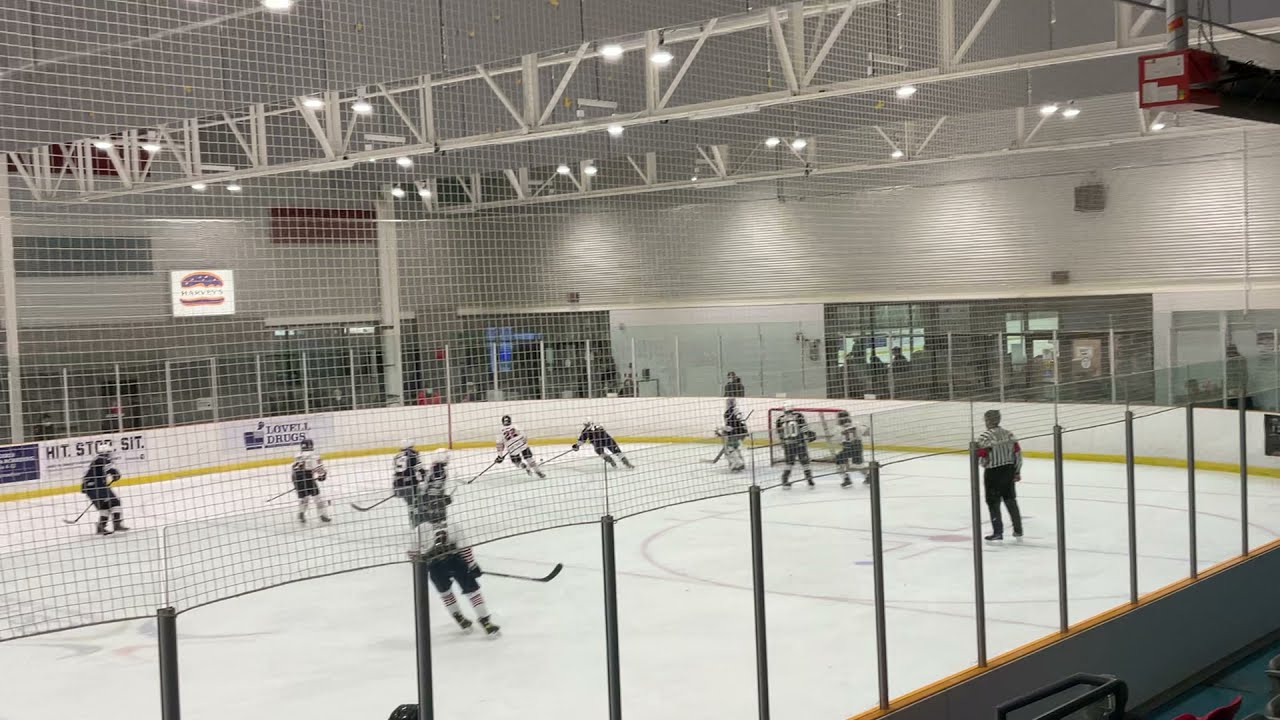This detailed color photograph captures an interior view of a hockey rink, taken from the stands in landscape orientation. The perspective is from a slightly elevated position, looking down towards the ice. The image prominently features several players in action, with one referee in a traditional black and white striped uniform standing to the right of the center, facing away from the viewer. The players appear to be children, with one team wearing black jerseys and black pants, and the opposing team in white jerseys with black pants.

In the lower right corner of the image, part of the concrete barrier and the supporting posts with plexiglass panels are visible. To ensure audience safety, a mesh netting extends from the top of the plexiglass up to the ceiling, designed to catch any stray pucks. 

Overhead lights illuminate the rink, and a variety of indistinguishable advertisements line the walls around the playing area. The realism of the photograph captures the energy and structure of a live hockey game in progress.